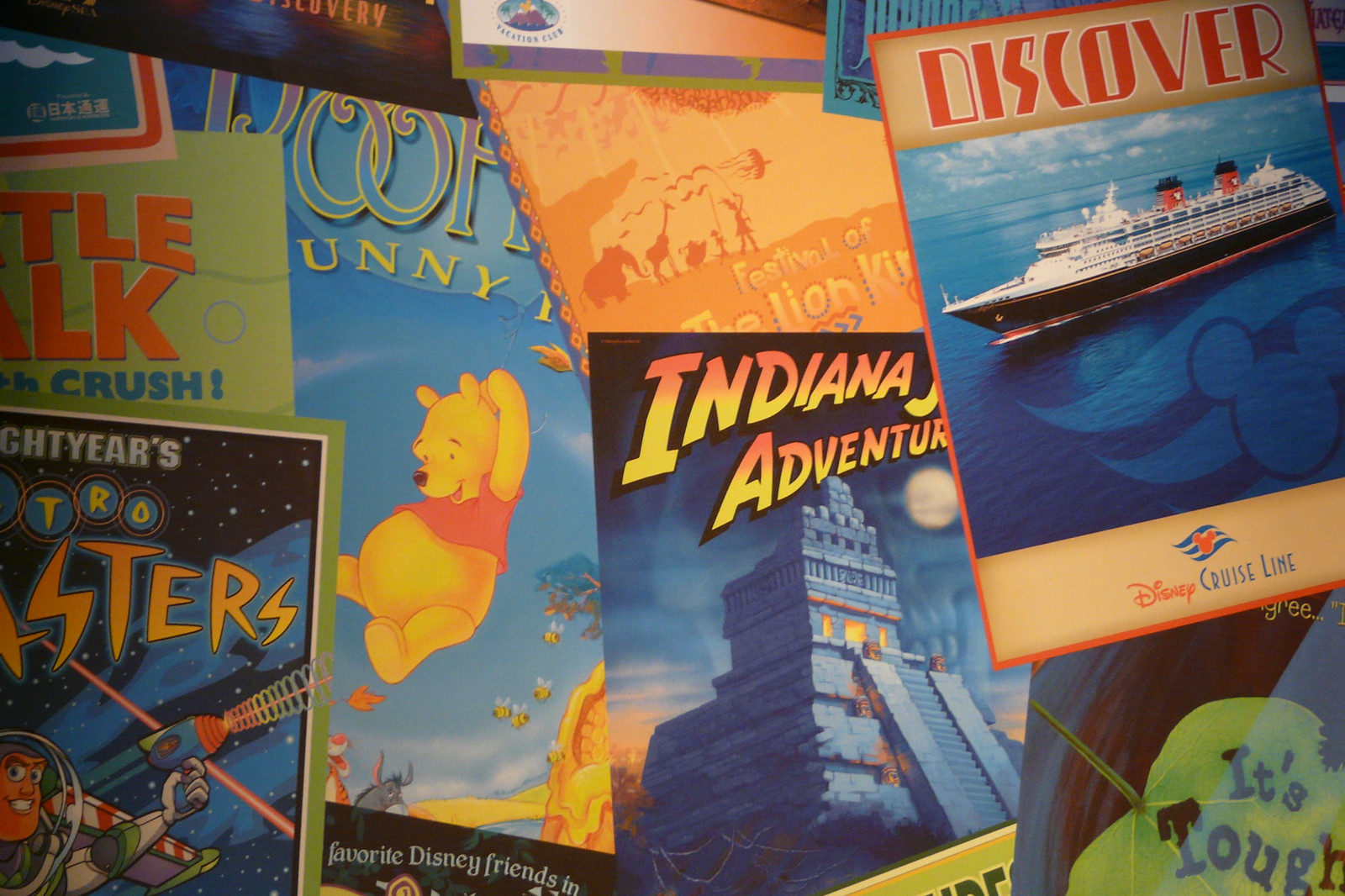This image showcases a wide rectangular collage of several vibrant and colorful posters, overlapping each other in a visually striking display. Prominently featured in the top right corner is a vertically-aligned, slightly tilted poster advertising Disney Cruise Line; it has the word "Discover" in bright orange font at the top and an image of a cruise ship sailing on blue waters, with the text "Disney Cruise Line" in orange and blue beneath. Just below and to the left, there is another poster for Indiana Jones, depicting a blue temple against a night sky backdrop. Above this, a charming image of Winnie the Pooh with his yellow fur and orange shirt is set against a clear blue sky. In the bottom left corner, Buzz Lightyear makes an appearance, enhancing the Disney-themed assortment. The rest of the posters share a similar bright color scheme, contributing to the cohesive yet dynamic patchwork of Disney-themed advertising.